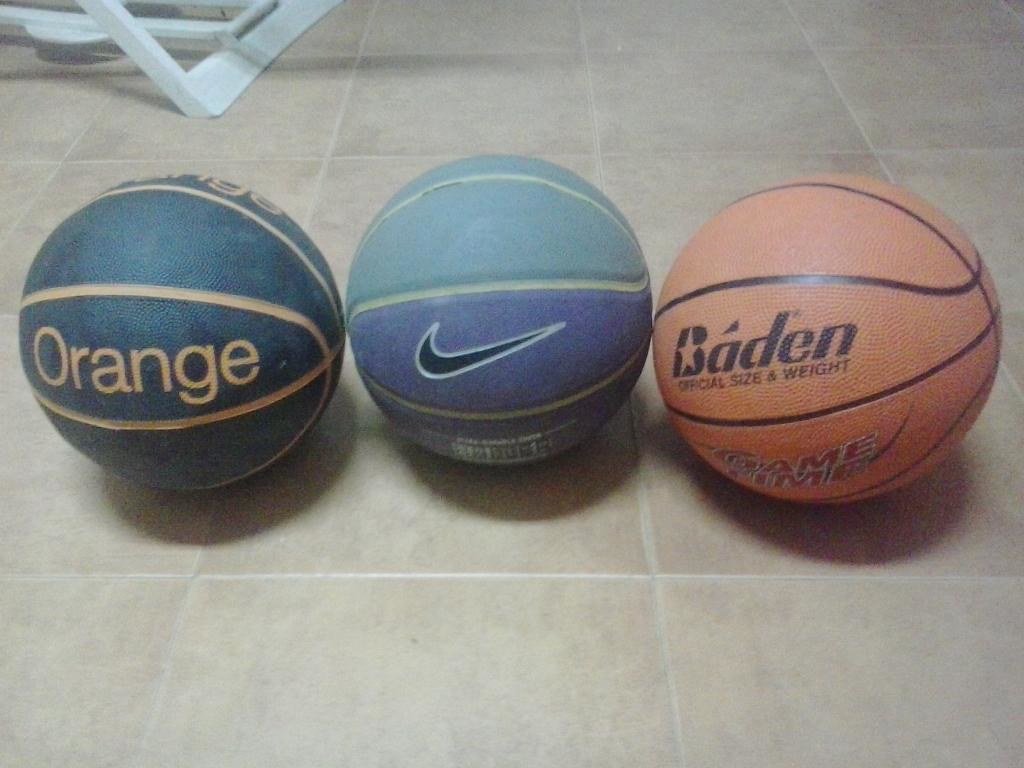This photograph depicts three distinct basketballs positioned on a beige tiled surface with white grouting between the tiles. From left to right, the first basketball is dark blue with orange stripes and features the word "ORANGE" prominently printed in orange letters. The middle basketball displays a blend of teal and royal blue colors with pea green lines and is adorned with a black Nike swoosh. The basketball on the right is the traditional orange ball with black stripes, bearing the brand name "Baden" in black text, along with "OFFICIAL SIZE AND WEIGHT" and partially visible red text that likely reads "Game Time". In the upper left corner of the image, the leg of a white plastic chair is partially visible, adding a subtle element to the scene, which might be set on a kitchen floor.